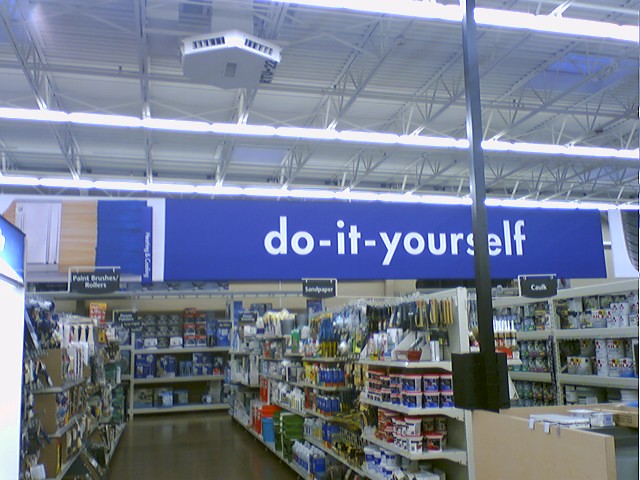The image captures the interior of a large hardware store, characterized by an open ceiling displaying a network of white steel girders and multiple horizontal air ducts. Dominating the upper background is a large rectangular blue banner that prominently reads "Do It Yourself" in white letters. The store is organized into several aisles labeled with black signs indicating various home improvement categories such as paint, paint brushes, rollers, sandpaper, and caulk.

The flooring is a shiny dark gray, adding a sleek contrast to the vibrant shelves lined with a variety of products. Notably, the bottom right corner of the image features a desk, suggesting an area for customer service or consultations. The aisles are well-stocked with an array of home improvement items, including cans of paint, tubes of caulk, different types of sandpaper, and paint rollers, which are visibly arranged on the neatly organized shelves. The detailed layout and clear signage aim to guide customers through their DIY shopping experience efficiently.